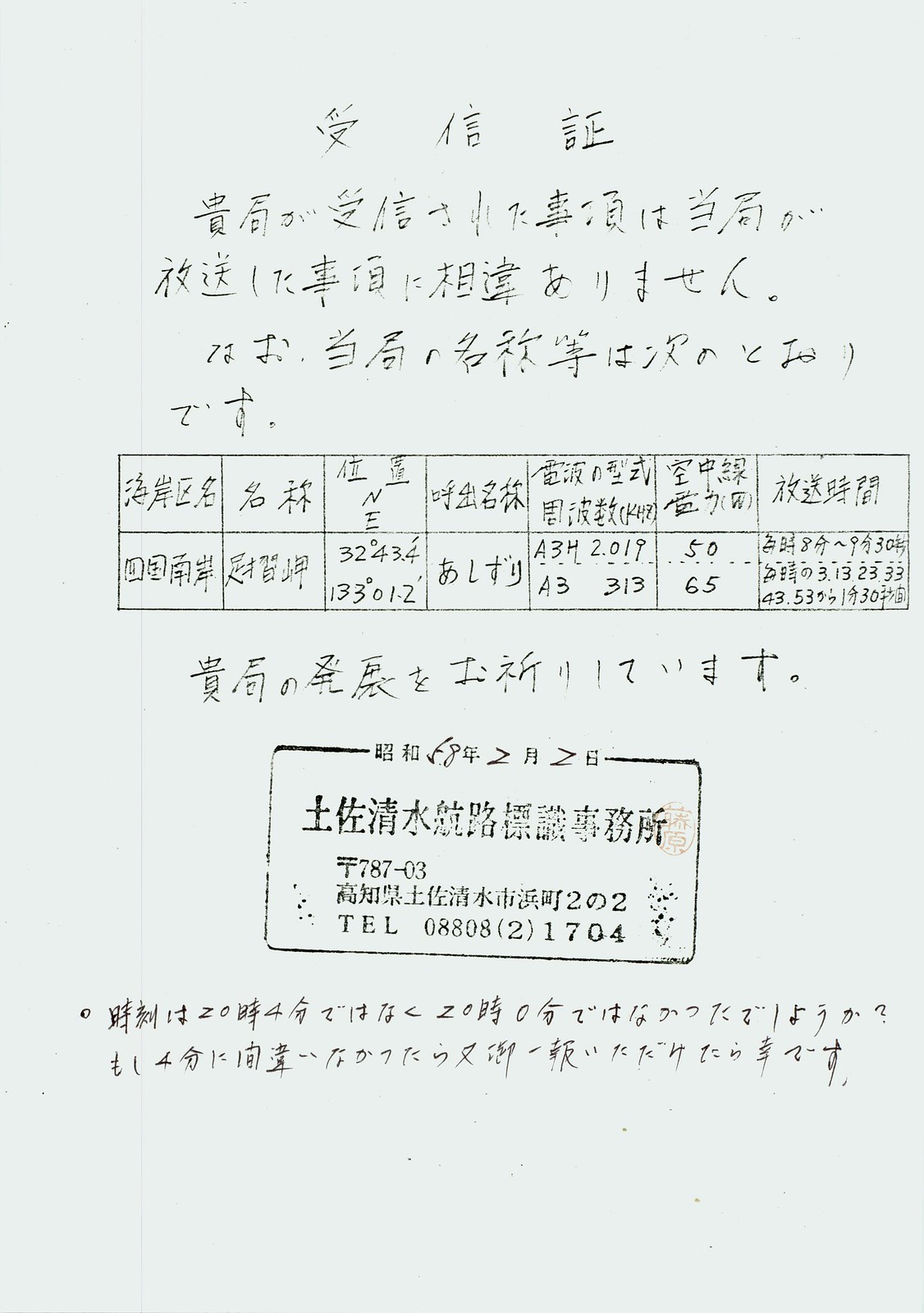The image shows an old, possibly library-related card or document, that appears to be written in either Japanese or Chinese, featuring a mix of sentences or mathematical text at the top. The central section of the document includes a table or a box structure with two rows and seven columns, containing the number 787-03. Near the bottom of the card, there is a stamp and a telephone number: 0880821704. The card appears to be from an era before digital barcode systems were prevalent, as it lacks any barcode. There are no people in the image, and despite the worn look suggesting age, the exact purpose of the card remains unclear.